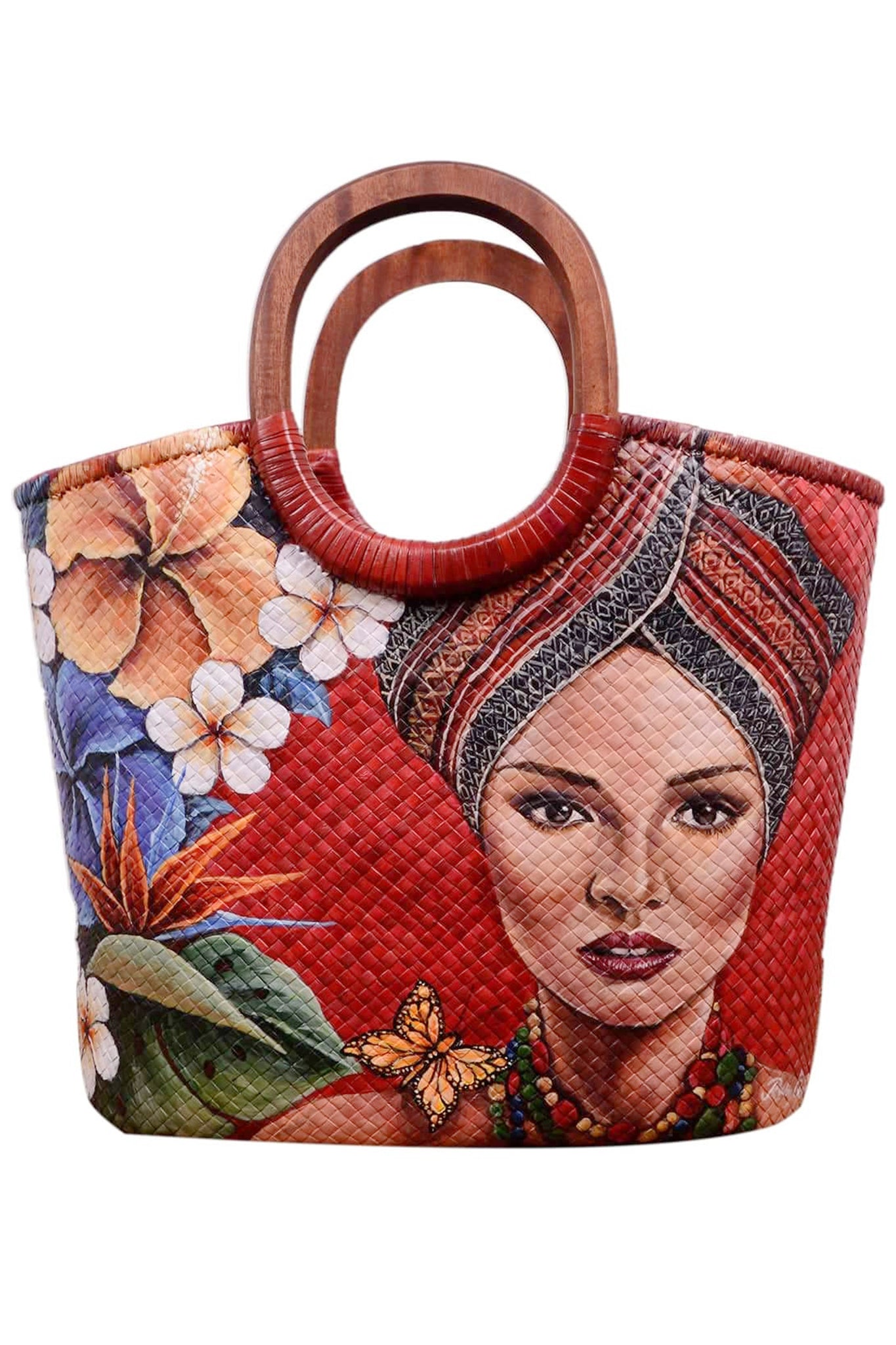This close-up color photograph showcases a meticulously crafted, hand-woven handbag set against a plain white background, likely intended for a catalog or online sale. The handbag, approximately 12 inches tall and 12 inches wide, is predominantly red and constructed from a sturdy material, possibly bamboo or a similar fabric.

It features two circular wooden handles, attached with red stitching, enhancing both the bag's aesthetic and utility. The open-top, square-shaped handbag is adorned with a vibrant, detailed print on its front.

Dominating the design is an image of a woman with dark eyes and brown skin, her head wrapped in a striking blue, red, and black headdress. She wears multiple bead necklaces and boasts red lipstick. A monarch butterfly perches delicately on her shoulder.

To the left of the woman's portrait, an array of tropical flowers, including a bird of paradise in orange, purple, and green, white flowers, a prominent orange flower, purple flowers, and green leaves with spiky red leaves, cascade from the lower left corner to the upper right, creating a rich and colorful contrast against the vivid red background of the handbag.